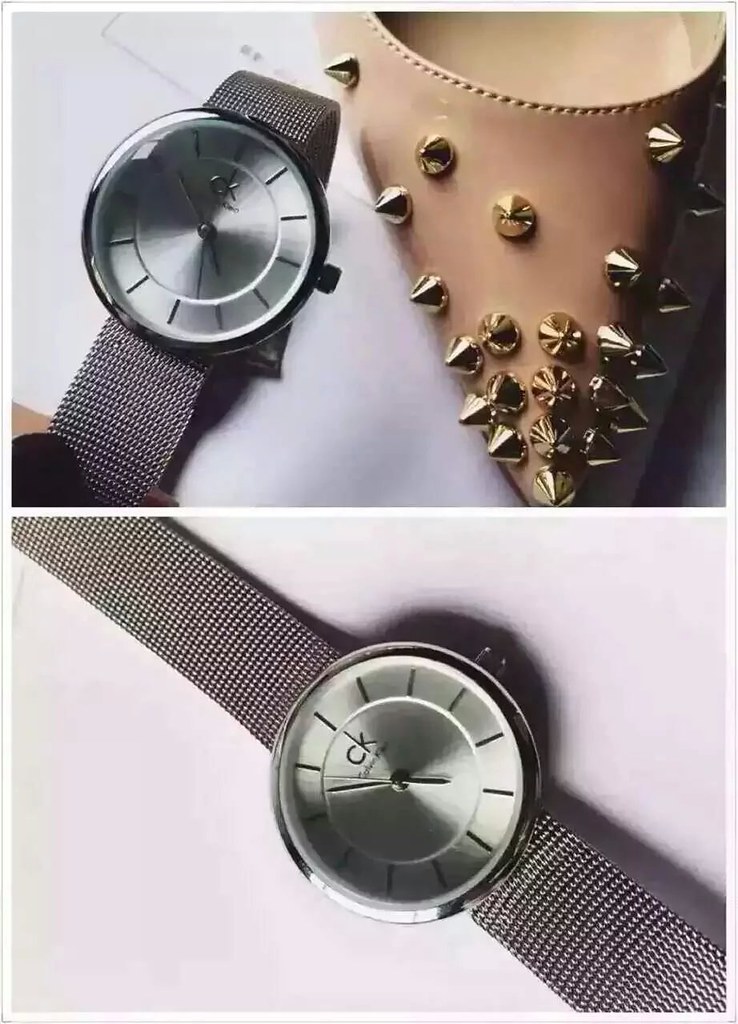The image is split into two sections, each showcasing distinct items against a clean, white background. 

In the top section, a close-up view highlights a stylish assembly of a silver watch and a light brown shoe. The watch, prominently displayed against the plain background, features a chainmail-like strap and a large silver watch face emblazoned with the initials "KC," presumably for Calvin Klein. The bezel appears to be either silver or black, adding a sophisticated touch to the timepiece. Positioned to the right, the shoe—light brown with a hint of a pinkish undertone—boasts an array of gold spikes, reminiscent of Louboutin’s iconic designs.

The bottom section offers an expanded view of the same watch, again set against a white backdrop. This shot allows for a more detailed look at the chainmail-like band, confirming its silver hue. The watch face remains the focal point, displaying the "KC" initials prominently in the center, underscoring the Calvin Klein branding.

This caption extensively details each element, providing a thorough visual description of the items showcased in the composed image.